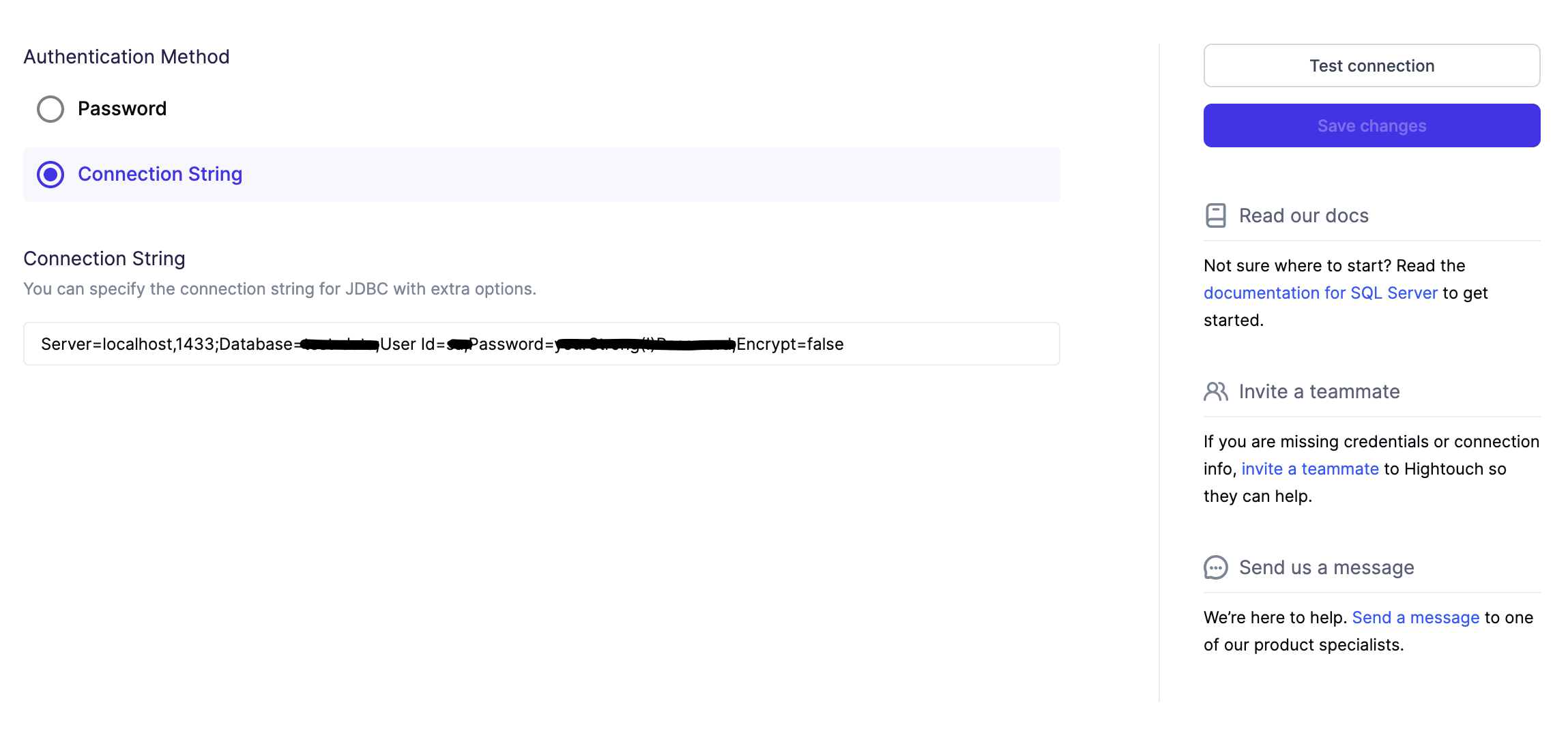This landscape-format color screenshot captures a functional user interface for setting up an authentication method. The design is straightforward and utilitarian, focused solely on functionality rather than aesthetics. At the top, a section titled "Authentication Method" allows the user to choose between "Password" and "Connection String," with the "Connection String" option selected. Directly below, a descriptive text permits the specification of a JDBC connection string along with additional options.

The image features extensive code detailing the connection string, with entries like "server=localhost,1433," among others, indicating server and port configurations. To the right, actionable buttons labeled "Test Connection" and "Save Changes" are visible. Further guidance is provided through hyperlinks in blue text, offering access to SQL server documentation for those needing assistance.

Additionally, there is a prompt to invite a teammate to HiTouch if credentials or connection information are missing. Another section encourages users to reach out to product specialists for further help, with a message-sending option for additional support. The background is predominantly white, with black text providing clear readability and blue hyperlinks offering easy access to further resources.